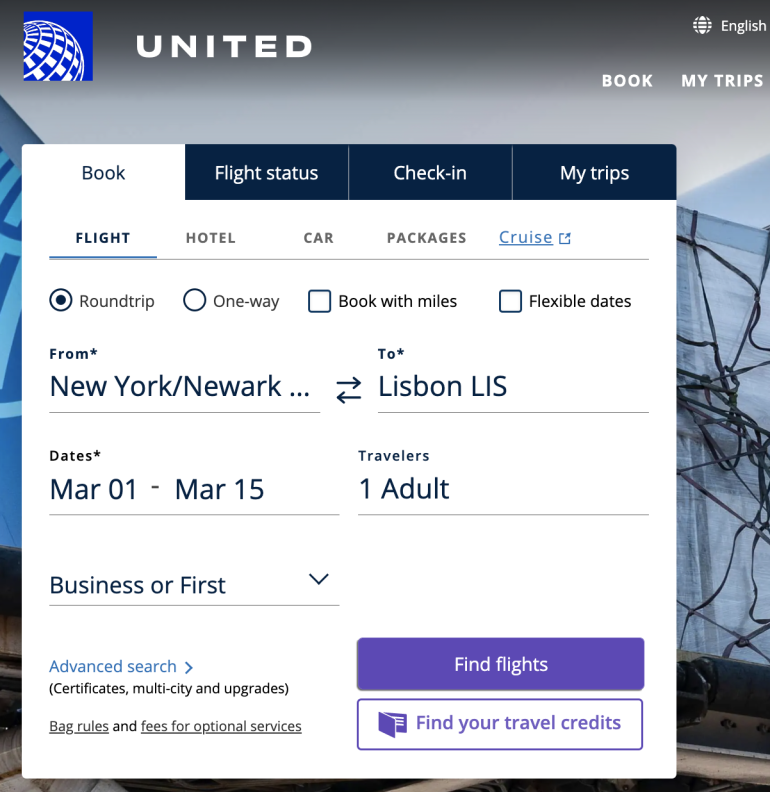The image displays a detailed user interface for booking travel on an airline website. The primary background is a gray hue, and along the left side, there is a section with a blue square that features illustrations of planets, suggesting a sense of exploration and travel. The interface is designed in English.

On the right side, there is a menu listing various travel options: "My Trips," "Flight Status," and "Check-In." The central booking section includes options for booking flights, hotels, cars, packages, and cruises. Users can choose between "Round-Trip" (which is selected) and "One-Way" (which is not selected), with additional options to book with miles or search for flexible dates.

The specific travel route listed is from New York/Newark to Lisbon (LIS), with travel dates from March 1st to March 15th. The travel class listed is "Business or First," and there are options for advanced search, certificates, multi-city trips, upgrades, bag rules, and fees for optional services.

A prominent purple bar displays a "Find Flights" button, and there is a distinct section labeled "Find Your Travel Credits" indicated by a hollowed-out icon resembling a wallet. In the background, there appears to be a net, possibly indicating cargo or luggage transport, adding a dynamic, layered element to the overall interface.